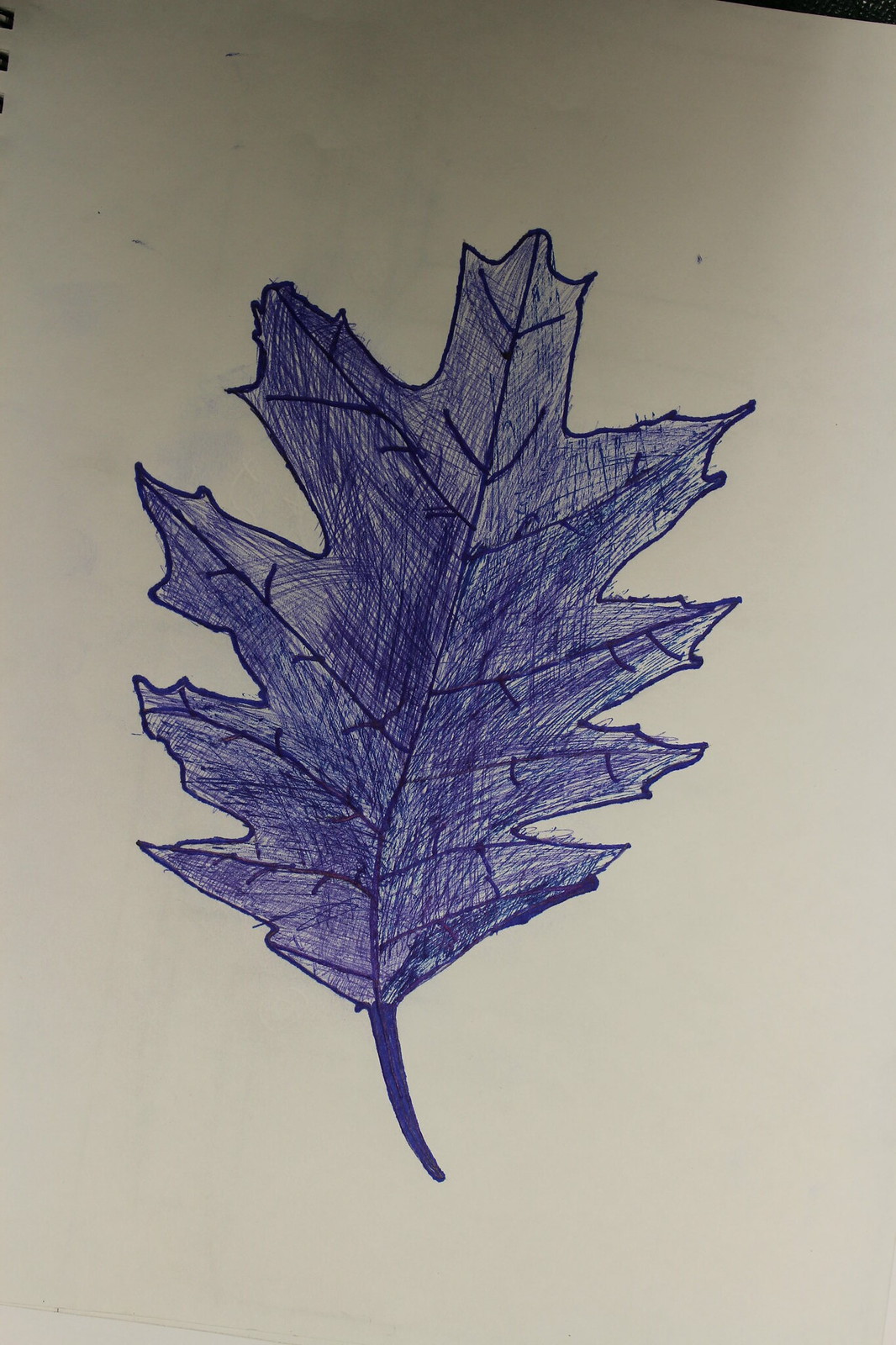This image features a detailed, hand-drawn illustration of a single leaf prominently centered on a plain white sheet of paper. The leaf itself is rendered in a blue hue, showcasing a clear central vein that runs vertically from the stem at the bottom to the pointed tip at the top. Offshooting from this central vein are several smaller veins extending towards the left and right, creating a natural, branching vein structure typical of a leaf. The leaf's edges are intricately drawn, tapering to sharp points on both the sides and the apex. The background behind the leaf drawing is also white, marred only by a few subtle blue marks scattered across the sheet, adding to the simplicity and focus of the composition. The overall effect is a minimalist yet striking study of botanical form in a monochromatic blue palette.